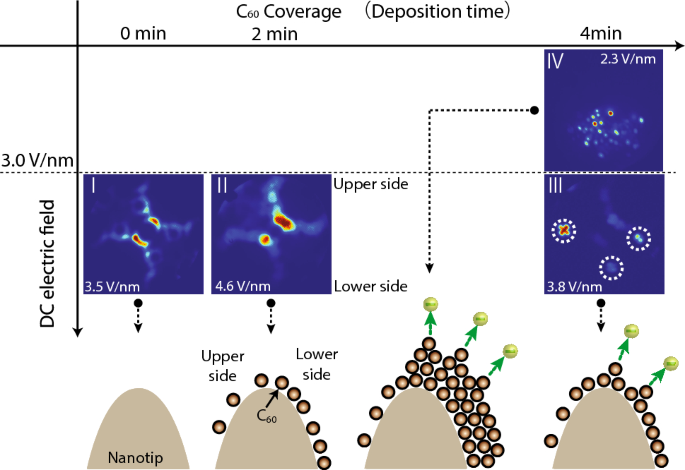The diagram depicts a graphical representation of a DC electric field measured in volts and minutes. In the top left corner, a black arrow points downward, intersecting a horizontal black line that stretches across the screen, creating a grid-like appearance. The diagram starts at "0 min" on the left, moves through "2 min" with the label "C60 coverage (deposition time)," and ends at "4 min" close to the right edge.

Above the horizontal line are two blue, x-ray style images featuring yellow and white spots, with annotations that indicate voltage levels of "2.3V/nm" and "3.8V/nm." The downward arrow alongside the depiction signals the direction of the DC electric field.

Below the dotted horizontal line positioned about two-thirds down the screen, the right side hosts two small images with yellow centers. Further down are a series of four side-by-side panels illustrating nanoscale interactions. 

- The first panel shows a smooth beige hill labeled "Nano Tip."
- The second panel features approximately ten round brown balls rolling over and around a similar hill.
- The third panel displays three rows of approximately thirty round brown balls stacked on top of each other, with green arrows pointing at three small brown balls.
- The fourth panel illustrates a line of around ten round brown balls, with one elevated just past the peak, accompanied by green arrows pointing to small white balls. 

This detailed and annotated diagram visually portrays the application of a DC electric field and associated changes over time and space at the nanoscale level.